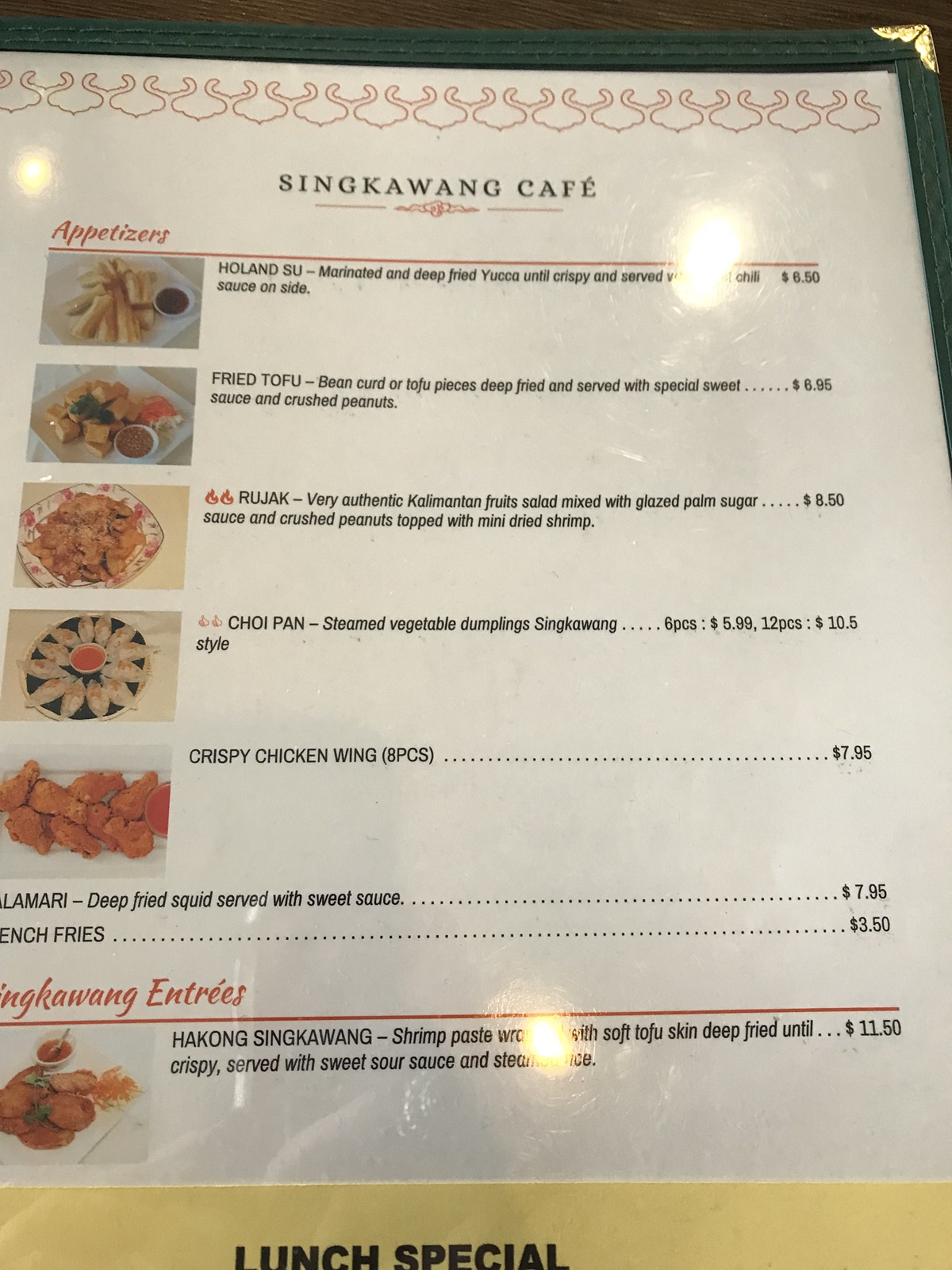The image depicts a laminated menu that is reflecting light, creating bright spots in the top right and left corners, as well as at the bottom. At the very top of the menu, there are hooks for hanging. On the left side, the appetizers section is visible, listing an assortment of dishes.

In the middle of the menu, there's a notable mention of "Holland," related to a marinated deep-fried yucca and tofu dish priced at $6.50. The menu also offers fried tofu, bean curd, or tofu pieces, which are deep-fried and served with a special sweet sauce and crushed peanuts for $6.95.

The right side of the menu features an entry labeled "Rootjacks," noted for its two flame symbols. The menu section includes an authentic Kalamata fruit salad mixed with black palm sugar, priced at $8.50. This salad is topped with sauce, crushed peanuts, and mini dried shrimp. Another dish called "Toy Pond" lists steamed vegetable dumplings, with prices of $6.60 and $5.99, or $10.50 for 12 pieces.

Additional menu items include boneless crispy chicken wings (8 pieces for $7.95), deep-fried calamari served with herbs and sweet sauce ($7.95), and French fries priced at $3.50. Other items listed are oranges, "Hot Gong," shrimp paste with soft tofu skin, bread and toast, crispies, herbs and sweet sauce, and steamed rice, priced at $11.50.

At the bottom of the menu, a yellow rectangle indicates a lunch special. The surrounding lawn and cafe setting, along with the reflected light on the laminated menu, complete the scene, suggesting a cozy dining environment.